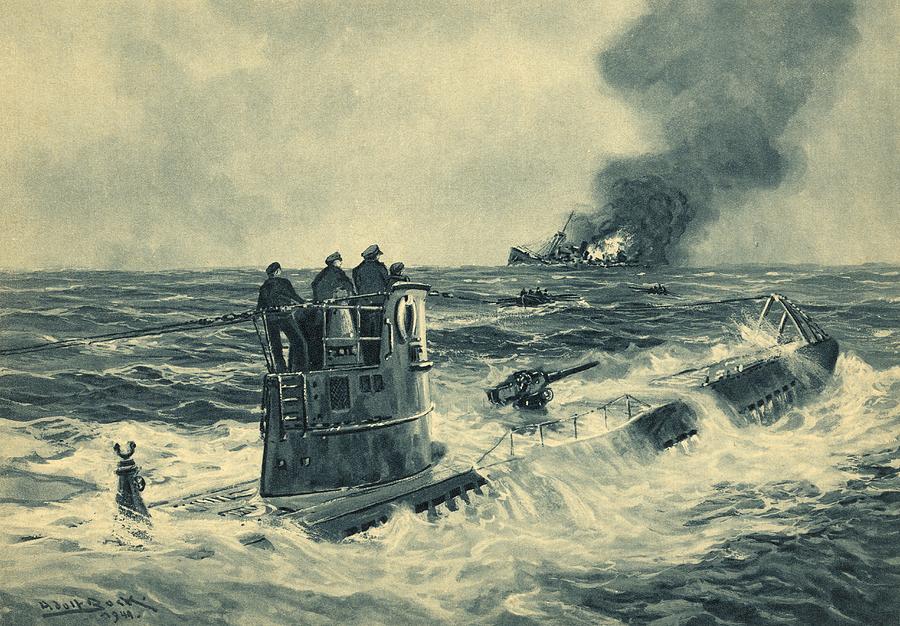This evocative blue-toned watercolor or painting, potentially signed "Hedelk Bach, 1949" in the lower left corner, captures a dramatic World War II naval scene. Dominated by turbulent, fire-lit seas with billowing black smoke, the painting likely depicts a submarine partially surfaced with its conning tower apparent. Four sailors, clad in caps and jackets, stand atop, intently staring at the horizon where a burning vessel is visible and ominously sinking. Lifeboats with indistinguishable figures are seen rowing through the rough waters, possibly trying to reach safety. A deck gun is also visible on the submarine, contributing to the wartime narrative. The entire scene is rich with details of chaos and destruction, enhanced by the crashing waves and the stark contrast between the dark smoke and the otherwise monochromatic palette.